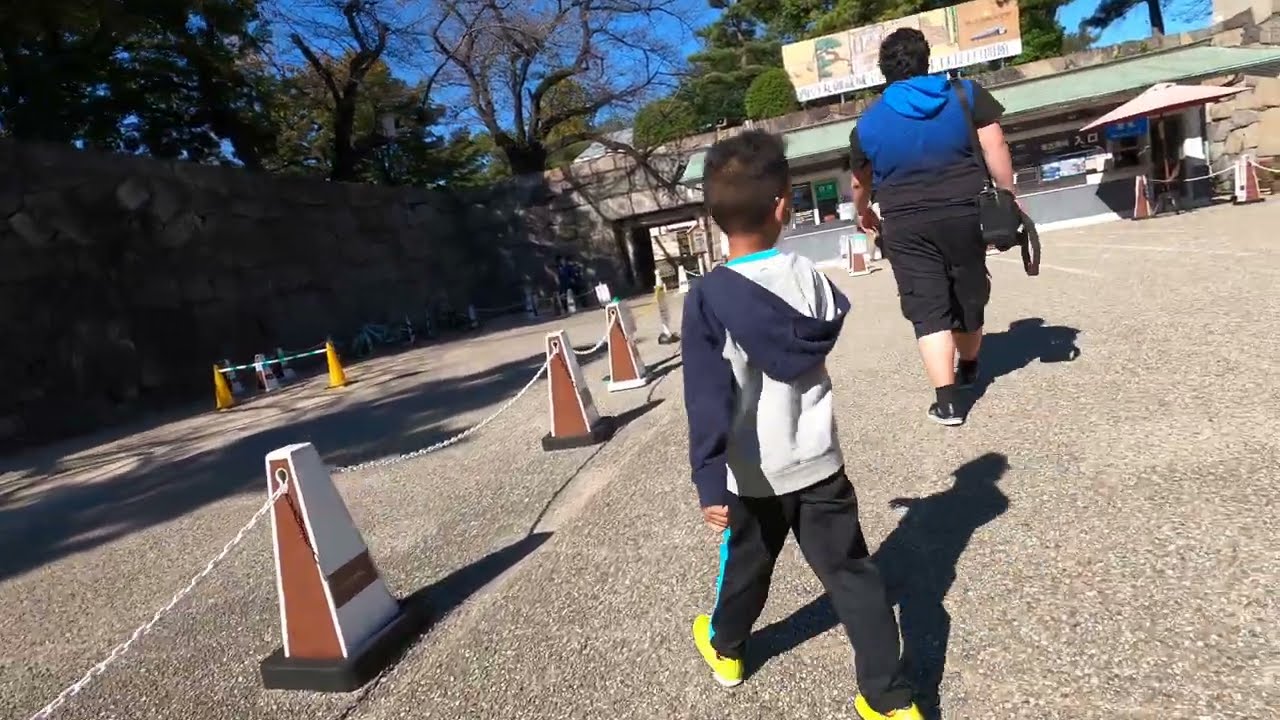In the horizontally aligned rectangular picture taken outdoors, a young child with darker skin and short, dark brown or black hair is slightly off-center in the foreground, walking away from the viewer. The child is dressed in a gray hooded sweatshirt with navy blue sleeves and a hood, black athletic pants, and striking yellow tennis shoes. He is following a slightly heavyset adult who wears a blue and black hooded short-sleeved shirt, black capri pants, and black tennis shoes. The adult has a bag slung over their right shoulder and seems to be holding something in their right hand. The duo is walking beside a series of safety cones connected by chains, which appear to section off this part of the parking lot.

The ground they walk on is a medium gray, and the area features white stripes just ahead of them, which seem to be part of the parking lot. They're heading towards a building that has a green awning out front. This older wood building sports windows and a door, with a kiosk-like arrangement resembling a ticket counter and a table with an umbrella near it. Above the building, a sign is visible but indistinct due to the distance in the image. A stone wall runs along the left side of the image, forming an archway near the business.

In the background, numerous trees are visible—some still bare, while others display green leaves. The clear blue sky peeks through the foliage, adding a calm ambiance to the scene. The overall composition suggests this area could be an entrance to an amusement park, zoo, or some kind of recreational business.